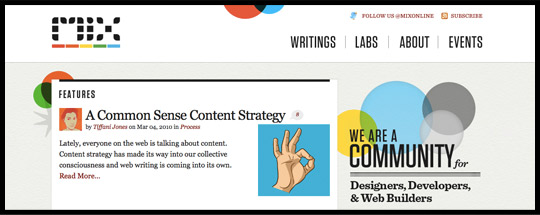This is a detailed screenshot of a website interface for MIX, featuring a dot matrix-style logo composed of five dashes in different colors: two orange, yellow, green, and blue. The logo is underlined by additional red and orange dashes. On the right side of the screenshot, there's a vertical navigation menu in all capital letters, listing the following options: "WRITINGS," "LABS," "ABOUT," and "EVENTS," separated by grey vertical bars. The text is displayed in black.

Above this menu, there is a Twitter icon with a prompt, "Follow us at MixOnline." Below that, there is an option to "Subscribe to their RSS feed." 

The background features a series of semi-translucent colored circles overlapping one another on a beige backdrop, creating a layered effect. In the bottom right section of the screenshot, large prominent text declares, "We are a COMMUNITY," highlighting the intended audience of designers, developers, and web builders.

On the left side of the screenshot, there is an overlay popup window with a black top bar labeled "FEATURES." This area includes a graphic representation of a face and a section titled "A Common Sense Content Strategy by [unreadable name], March 4th, 2010, in Process." Below this title is a snippet of text discussing the increasing importance of content strategy on the web, stating, "Lately everyone on the web is talking about content. Content strategy has made its way into our collective consciousness, and writing is coming into its own." The section ends with a red "Read more..." link.

Adjacent to this text snippet is a small graphic of someone making an "okay" sign, illustrated against a blue background.